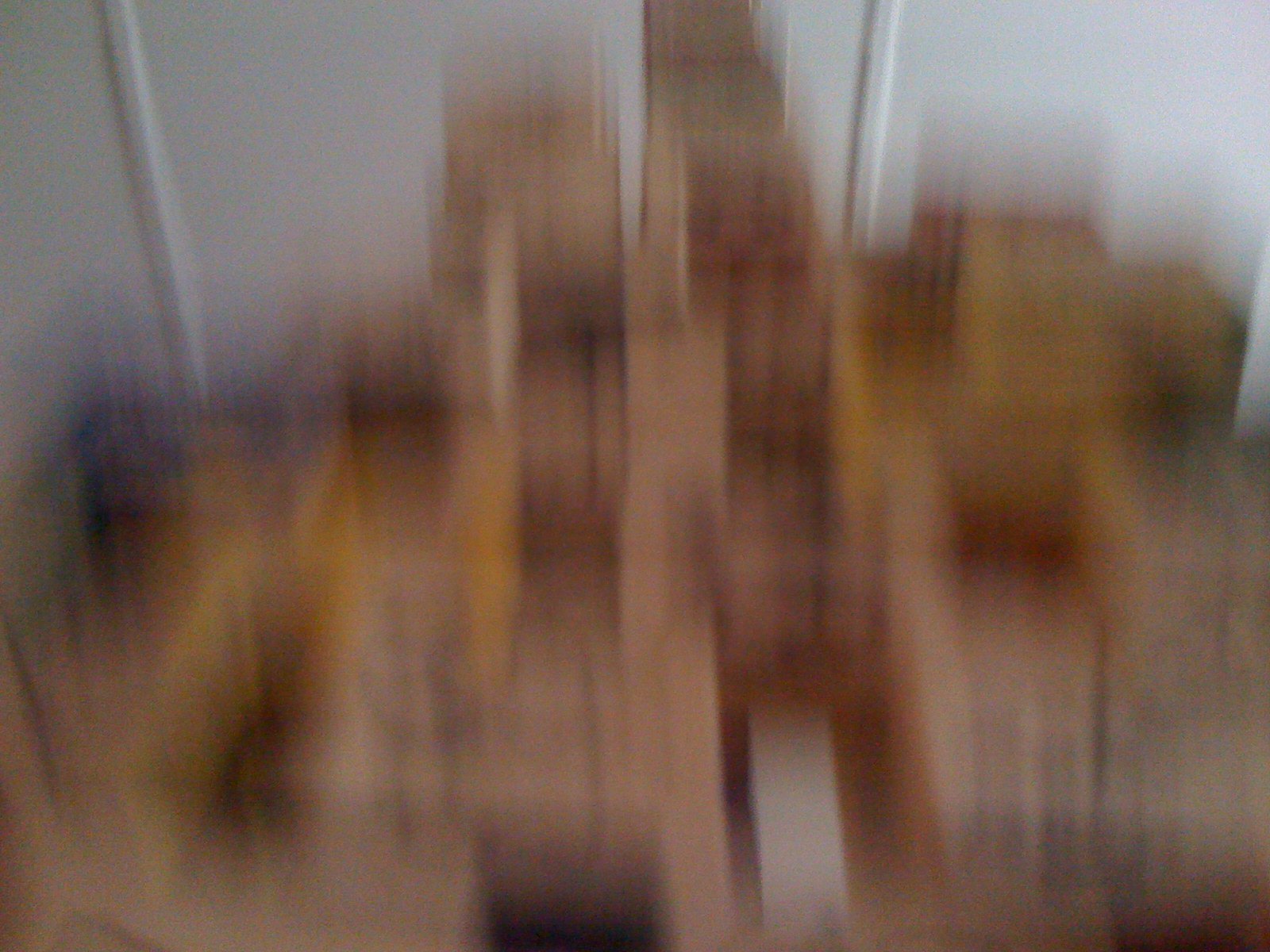This photograph is profoundly out-of-focus, characterized by a strong vertical blur, suggesting the camera or device was in motion, possibly falling, at the moment of capture. The scene appears to depict a cluttered floor with several cardboard boxes of varying conditions. Among the closest boxes, one is notably open, revealing a white object inside, which could be a piece of paper or a strip. Further back, other boxes are both stacked and open, creating a sense of disarray. The backdrop is a plain white wall, providing a blank contrast to the chaotic foreground.